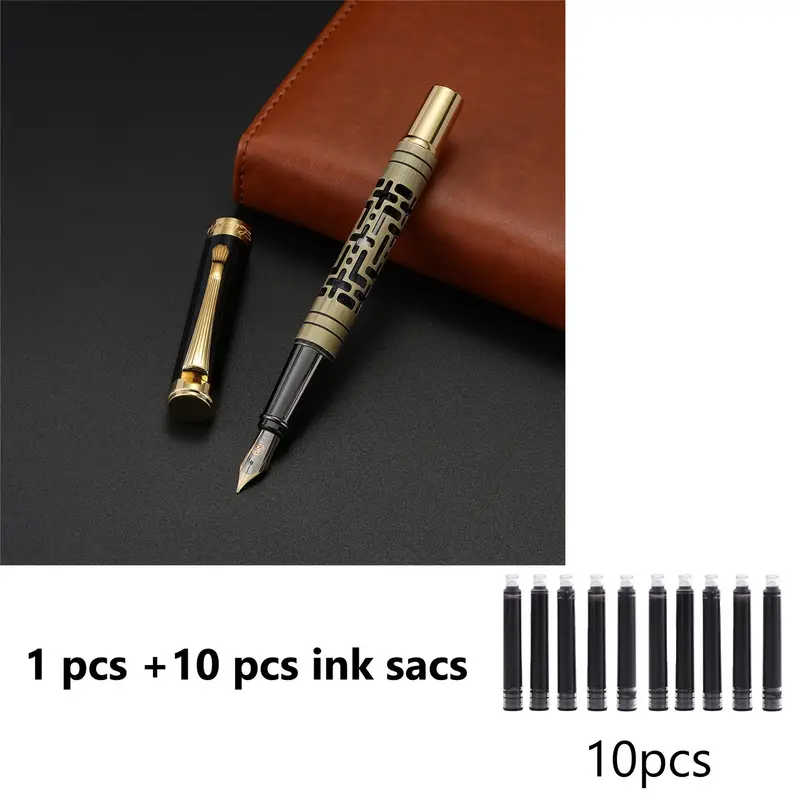The meticulously captured photograph showcases a high-quality fountain pen, predominantly featuring a sophisticated gold and black pattern. The pen, with a brass body transitioning to a black front end, is neatly displayed on a rich, brown leather book with visible stitching along the top edge, all set against a smooth, black tabletop. Emphasizing its luxurious details, the pen’s cap is adorned with a gold overlay on a black main body, providing a striking contrast. The product photo, characterized by professional lighting devoid of any reflections or highlights, points to a top-tier advertising effort. Below the pen and book, a banner displays the text "one piece plus ten pieces ink sacks," accompanied by a genuine image of ten ink cartridges, each distinctly different, indicating the authenticity of the product display.